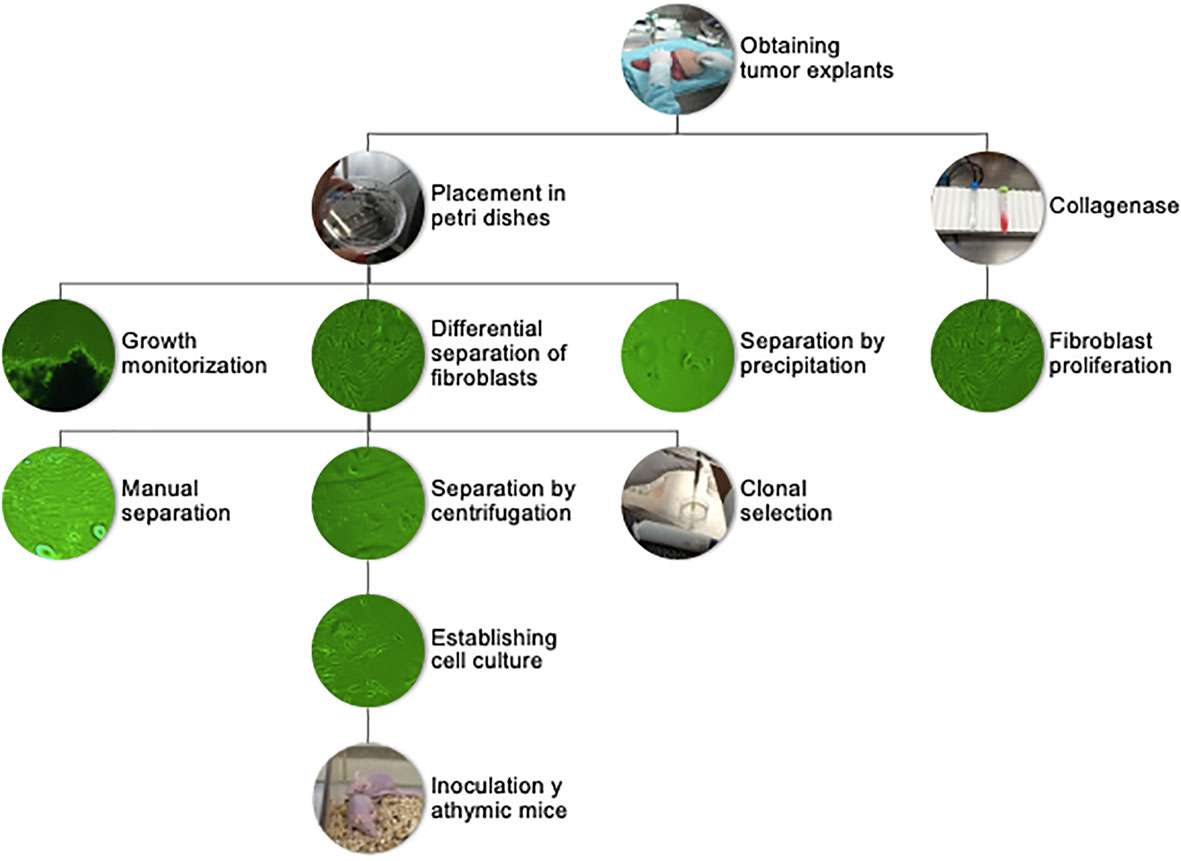This scientific diagram is a detailed flowchart illustrating the process of obtaining and cultivating tumor cells. At the top, it begins with "Obtaining Tumor Explants" as the central topic. This splits into two pathways: on the left, "Placement in Petri Dishes" and on the right, "Collagenase." Under the "Placement in Petri Dishes" pathway, there are three subsequent steps: "Growth Monitorization," "Differential Separation of Fibroblasts," and "Separation by Precipitation," each represented by green circles. These steps further break down into "Manual Separation," "Separation by Centrifugation," and "Clonal Selection" depicted in a white circle. Progressing further down this branch leads to "Establishing Cell Culture" and ultimately "Inoculation in Athymic Mice," illustrated with an image of mice in a container. Meanwhile, the "Collagenase" pathway progresses directly to "Fibroblast Proliferation." The combined processes are aimed at understanding tumor growth and cell culture techniques.